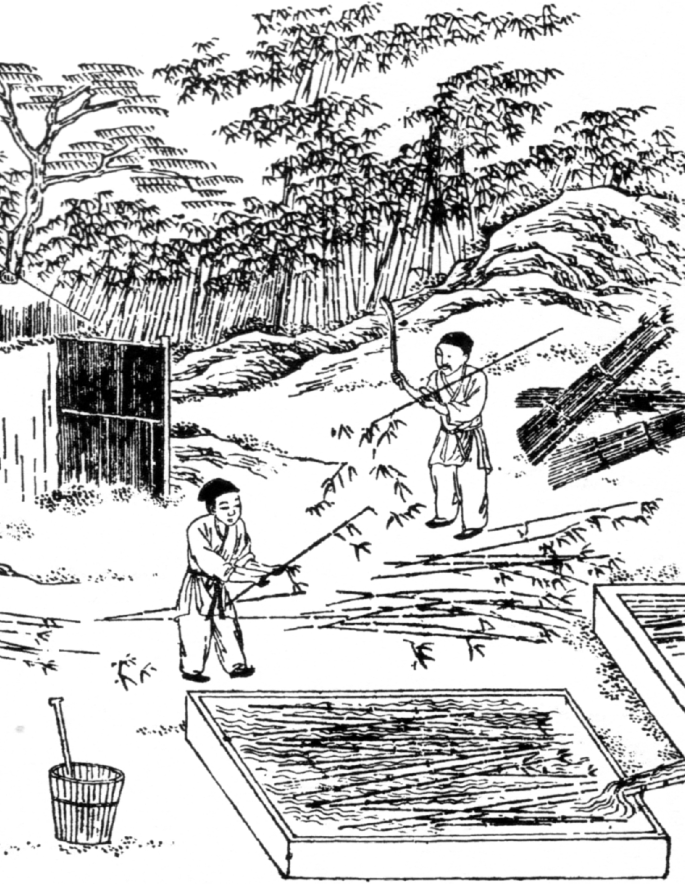The image is a detailed black and white line drawing depicting two laborers harvesting bamboo in an Oriental setting, likely a traditional farm or plantation. The focus is on the central figures, dressed in old-fashioned Eastern Asian work clothes. One laborer is wielding a knife or hatchet to chop the bamboo, while the other handles the stalks, removing leaves and preparing them for storage. They are placing the bamboo into a large rectangular bin or box, which appears to have water flowing into it from another similar container. To the lower left, there is a basket containing some sort of implement. The background features mounds of dirt, a fenced-in area with a small gate, and a stretch of bamboo running along a fence line. Additionally, visible are bundles of bamboo secured with straw and several storage structures made of bamboo. The illustration uses minimal shading and is mostly composed of clear outlines.